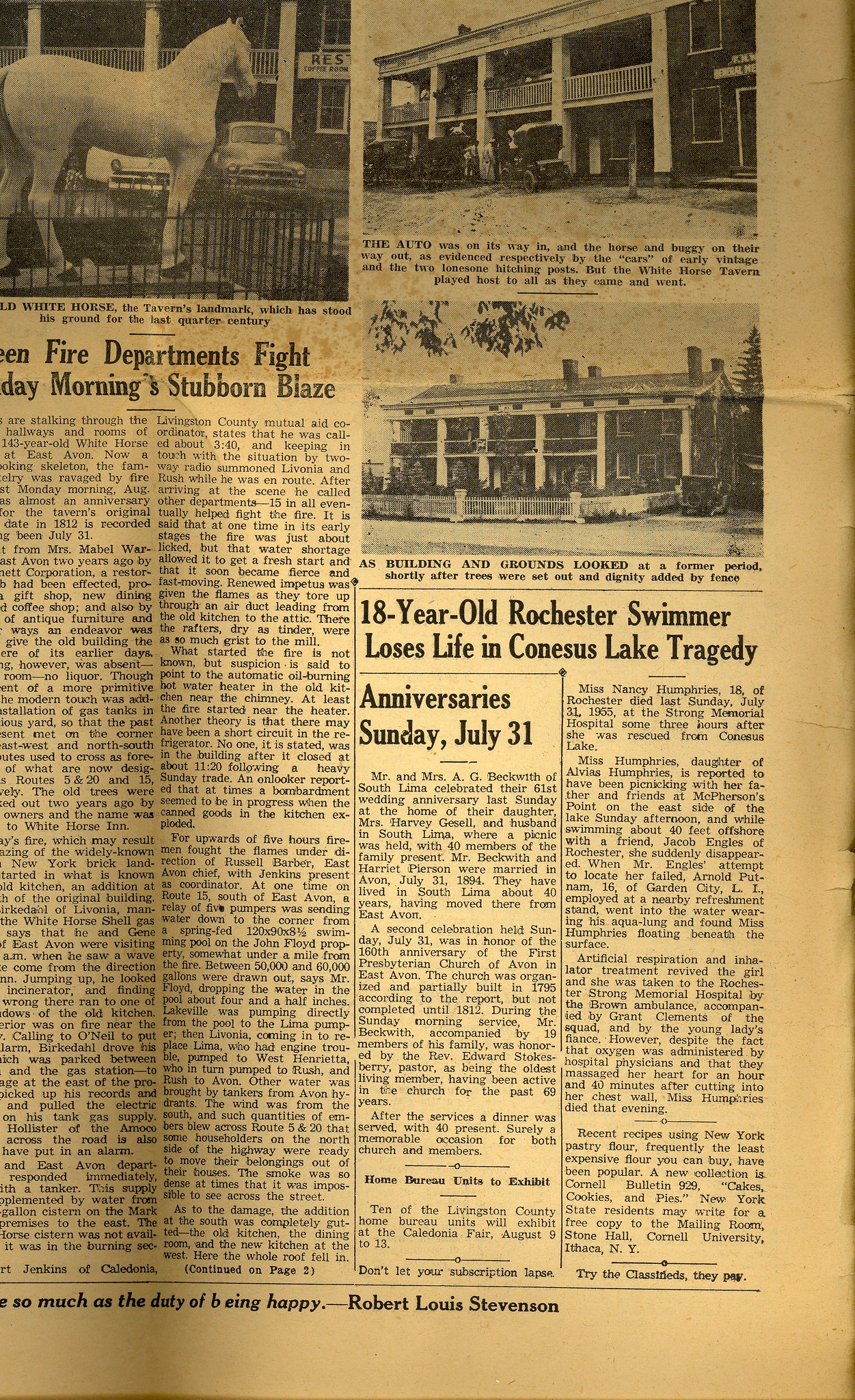The image is an aged, yellowed newspaper page, likely from the 1950s or 1960s, featuring multiple articles and photographs. Dominating the upper left-hand corner is a black and white photograph of a prominent horse statue captioned, "White Horse, the tavern's landmark, which has stood its ground for the last quarter century." Below this image is the headline, "Seven Fire Departments Fight Morning Stubborn Blaze," accompanied by two columns of text. To the right, another header reads, "18-Year-Old Rochester Swimmer Loses Life in Kenosha's Lake Tragedy," with a photograph of a large house's front porch with columns and another showing the entire house. Additional small text is present but illegible. The bottom section includes another headline, "Anniversaries for Sunday, July 31st," alongside the name "Robert Louis Stevenson." The newspaper is tattered, indicative of its considerable age and historical context.